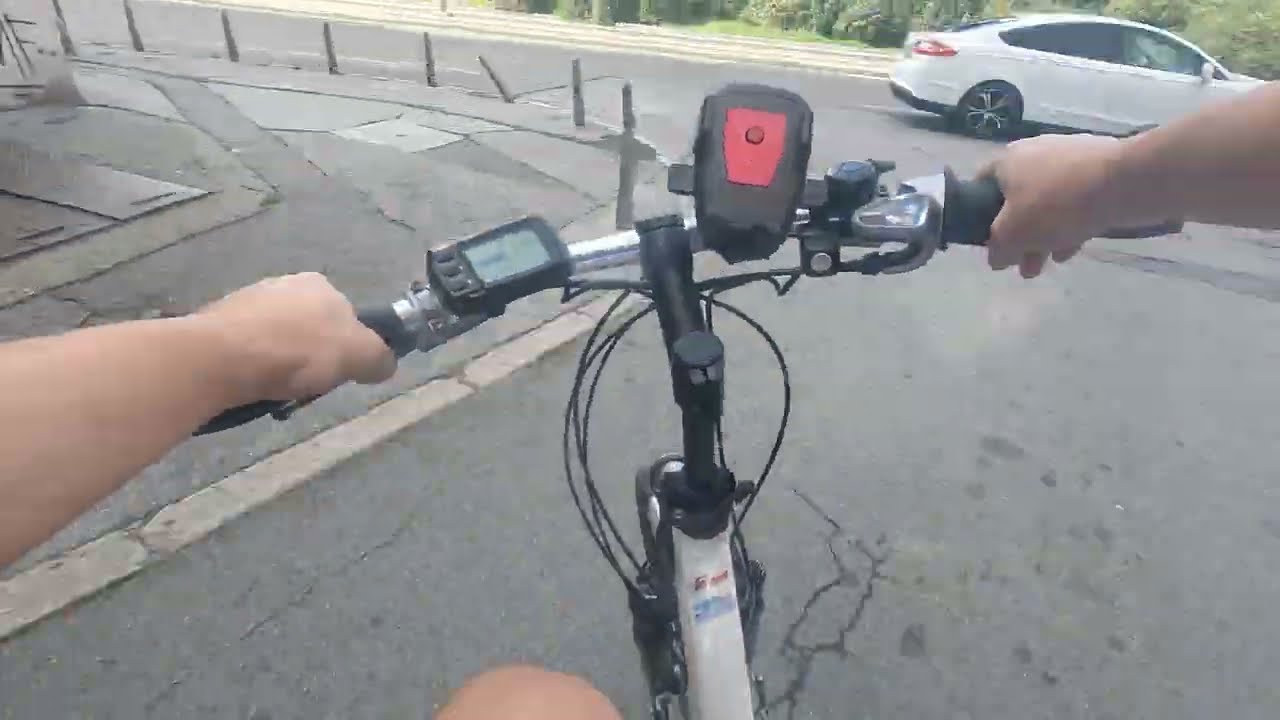The photograph captures a scene from the perspective of someone riding a bicycle on a paved, grey road. The view is from the rider's point of view, showing their hands gripping metallic black handlebars with attached instruments, likely a GPS and another device with a red cover. The bicycle itself is white with some black components visible. The front tire and part of the rider's knee can also be seen. The road ahead curves gently to the left, and in the top right of the image, a white car is either parked or driving from left to right. In the background towards the left, there is a sidewalk bordered by barriers, and beyond the road, a strip of green trees and grass provides a hint of nature against the grey asphalt.